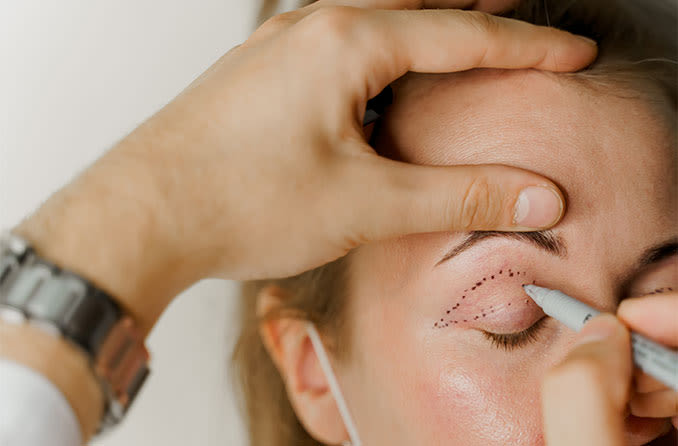In this close-up color photograph, a woman with dark, short hair and her eyes closed is being prepped for eyelid surgery, likely blepharoplasty. Her right eyelid is delicately marked with small dots by a gray, Sharpie-like marker, indicating areas for potential skin removal. A man's left hand, adorned with a silver metal-banded watch, gently lifts her right eyebrow. His right hand performs the careful marking. The woman is wearing a white mask, with a visible strap extending from her ear, though her face below the eyes is mostly obscured. The background is a stark white, focusing attention on the meticulous preparation procedure. The man appears to be wearing a white lab coat.